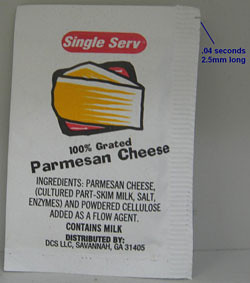The image showcases a small, single-serve packet of Parmesan cheese, similar to what one might receive at a pizzeria with a slice of pizza. The packet is rectangular with a vertical orientation and is primarily white. It features notable tear marks on the right-hand side, highlighted by a blue line with text indicating "0.04 seconds, 2.5 millimeters long." The packet prominently displays a red oval with a white background, marked with the text "single serve." 

Additionally, there is a red square with a black border situated below, containing an illustration of a yellow and white triangular cheese slice. This red square is labeled "100% grated Parmesan cheese." The listed ingredients are Parmesan cheese made from cultured part-skim milk, salt, enzymes, and powdered cellulose used as a flow agent. The packet also indicates that it contains milk and is distributed by DCS, LLC, located in Savannah, Georgia, 31405. The background behind the packet is plain white, which makes the packet's details stand out prominently.